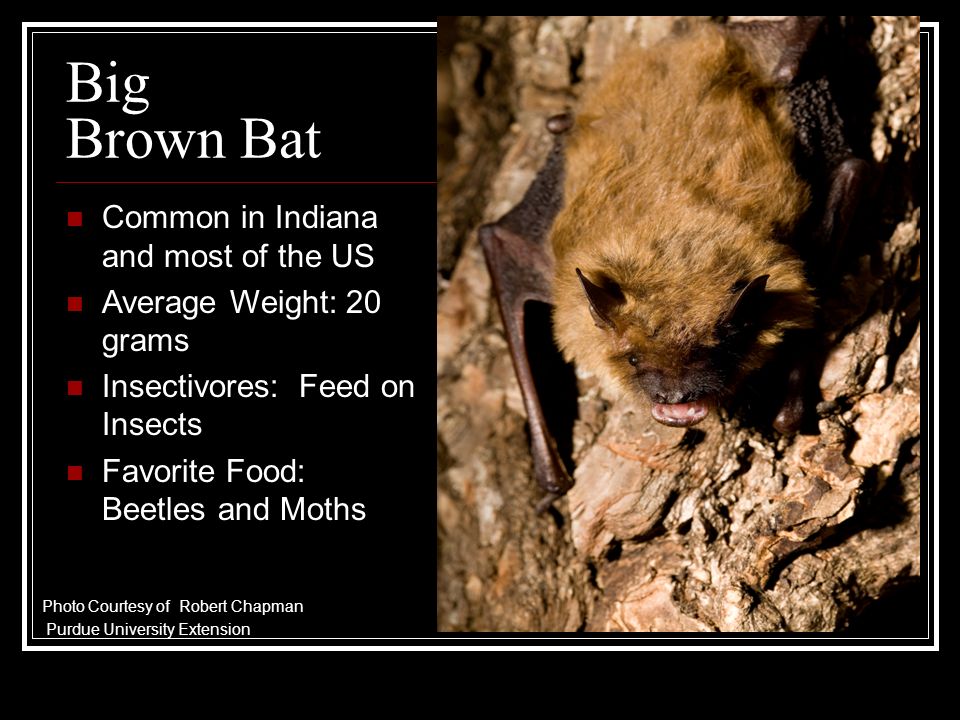The poster is a horizontal rectangular image with a black background and a white border just inside the edges. On the right side, there's a detailed, zoomed-in picture of a furry brown bat with pointy ears and dark eyes, its mouth open to reveal teeth. The bat is latched onto what appears to be tree bark. On the left side of the poster, large white text at the top reads "Big Brown Bat," followed by white text alongside red bullet points: "Common in Indiana and most of the U.S.", "Average weight, 20 grams," "Insectivores feed on insects," and "Favorite food, beetles and moths." The photo credit reads "Courtesy of Robert Chapman, Purdue University Extension."